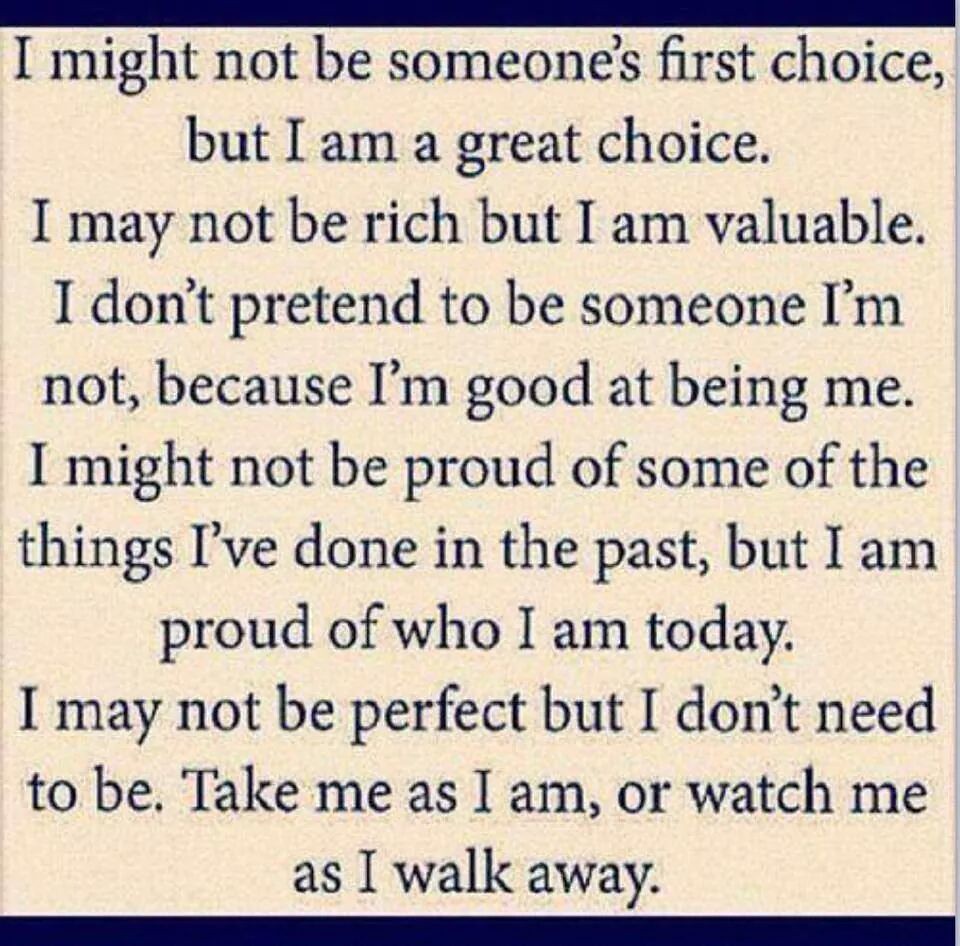The image features a motivational quote presented in dark blue, Times New Roman-like font on an off-white, cream-colored background marred by noticeable noise, suggesting low image quality. The text is neatly centered and extends nearly the entire width of the image. There are eleven lines, formatted with occasional indentation for emphasis. The quote reads: "I might not be someone's first choice, but I am a great choice. I may not be rich, but I am valuable. I don't pretend to be someone I'm not, because I'm good at being me. I might not be proud of some of the things I've done in the past, but I am proud of who I am today. I may not be perfect, but I don't need to be. Take me as I am, or watch me as I walk away." This text is vertically framed by thin, dark blue horizontal lines at the top and bottom, with very thin, almost imperceptible gray borders on the left and right sides, adding to the structured simplicity of the design.